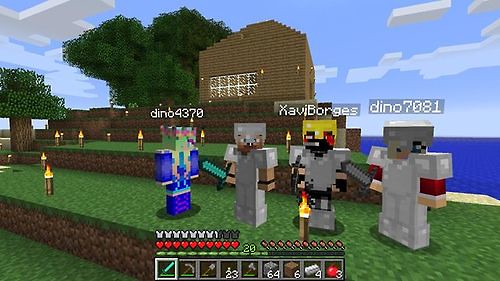The image depicts a nostalgic screenshot of an older, pixelated video game characterized by its blocky and non-realistic design. The scene comprises three layered, brick-like ledges, each adorned with brown edges and green tops, resembling grass. The background showcases a serene blue expanse, possibly an ocean or a large body of water, under a blue sky dotted with square, foam-like white clouds. On the left side of the image stands a tall tree, with an even larger one centrally placed, adding a touch of nature to the setting. Positioned behind the trees and ledges is a structure resembling a building, complete with windows.

The ledges are sporadically adorned with torches or similar objects protruding from the ground. The game characters, four robots with quirky user-assigned names such as Dino 7018, Zabby Borges, and Dino 4378, are dispersed across the levels. Notably, the bottom section of the image displays essential gameplay information: the count of missiles available and the number of lives remaining for the player.